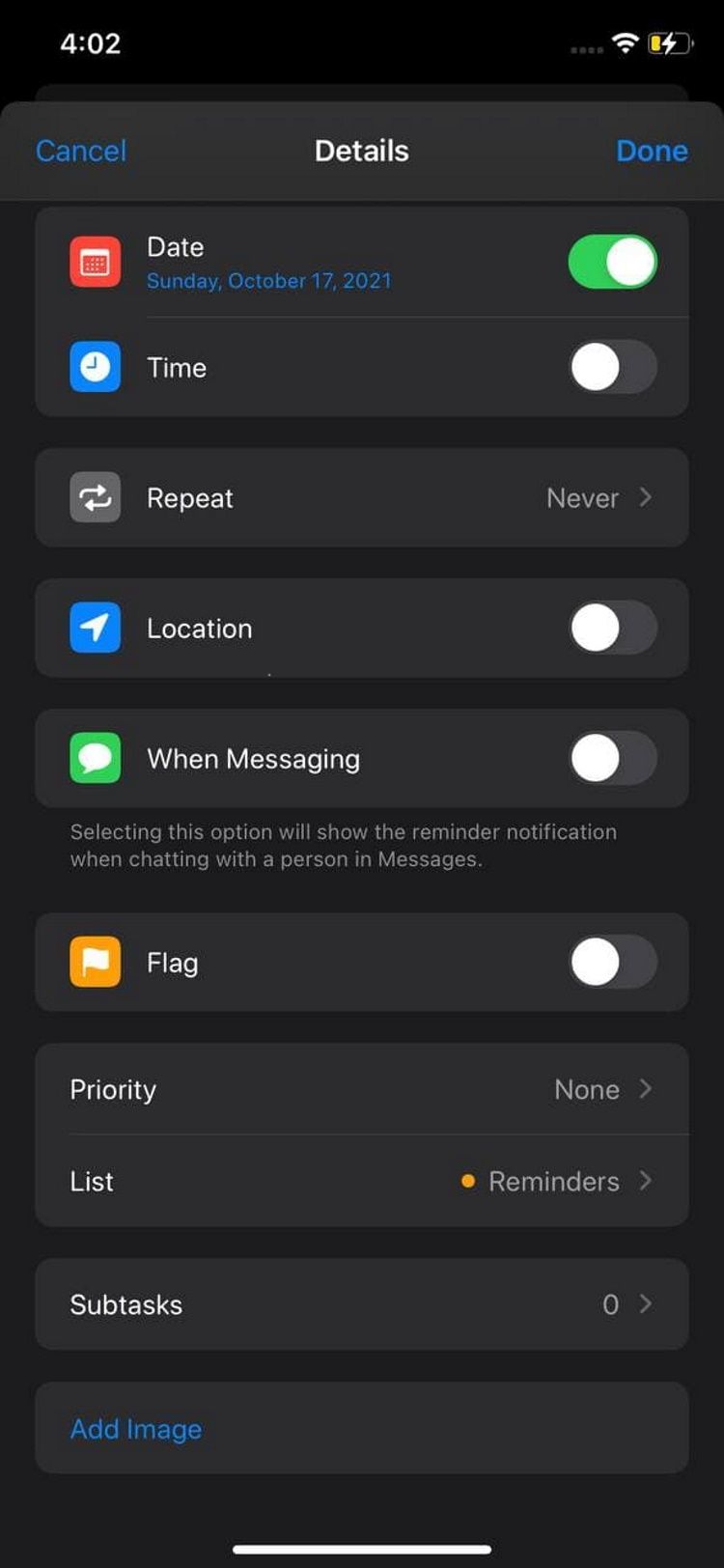The screenshot depicts a detailed view of a "Reminder" settings screen on an iPhone. In the top-left corner, the time is displayed as 4:02 PM, while the top-right corner shows no cellular signal bars, indicating that the device is connected to Wi-Fi. The battery icon reveals that the battery is about 20% charged and currently charging, as indicated by the charging symbol.

Centrally located on the screen is a pop-up window with "Cancel" on the left and "Done" on the right. The pop-up heading reads "Details." Below, several options and settings are listed:

- **Date:** Marked as Sunday, October 17, 2021, with a checkmark indicating it is selected.
- **Time:** Not enabled.
- **Repeat:** Set to "Never."
- **Location:** Not enabled.
- **When Messaging:** Option to show the reminder notification when chatting with someone in Messages, currently not enabled.
- **Flag:** Not enabled.
- **Priority:** Currently set to "None," with additional options available upon clicking.
- **List:** Set to "Reminders," with an accompanying orange dot suggesting newly available information or updates.
- **Subtasks:** Listed as zero, with more details accessible upon clicking.
- **Add Image:** An option available for adding an image to the reminder.

This detailed view provides a comprehensive breakdown of the reminder's configuration and the available settings options.